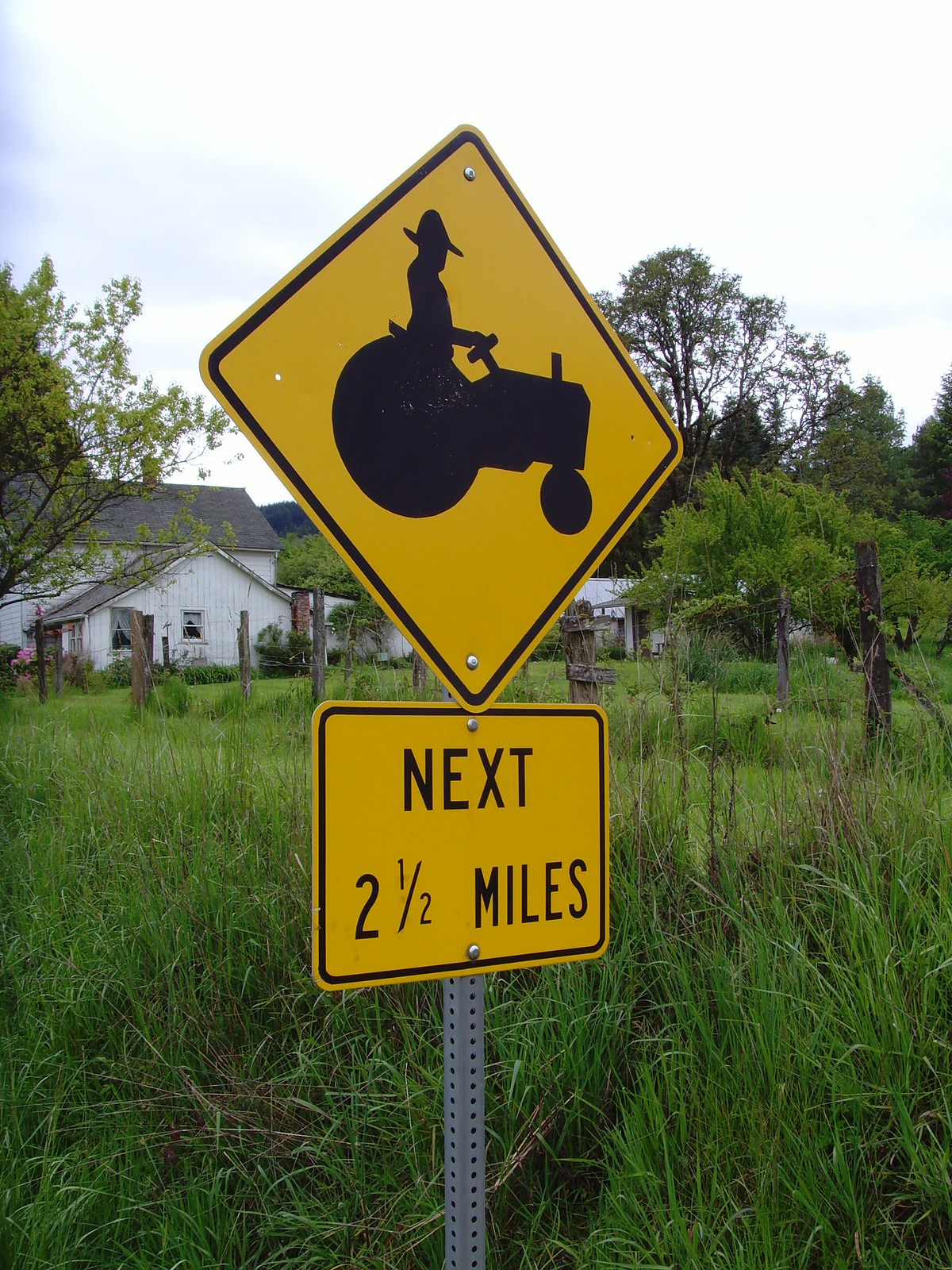In this outdoor image, a prominent yellow diamond-shaped street sign, topped with a silhouette of a man driving a tractor, is mounted on a gray metal post amidst an expansive yard filled with tall green and brown-tinged grasses. Beneath the tractor icon, a rectangular yellow sign with bold, black text reads, "NEXT 2 1/2 MILES." This information is secured with visible screws to the metal post. The setting exudes a tranquil, country-like atmosphere with various rural elements: wooden fence posts connected by wire, a white farmhouse with a gray roof, and another smaller structure nearby. The backdrop includes a scattering of leafy green trees and a predominantly white sky with a hint of blue. Scattered throughout the yard are additional posts, enhancing the rustic charm of the scene.